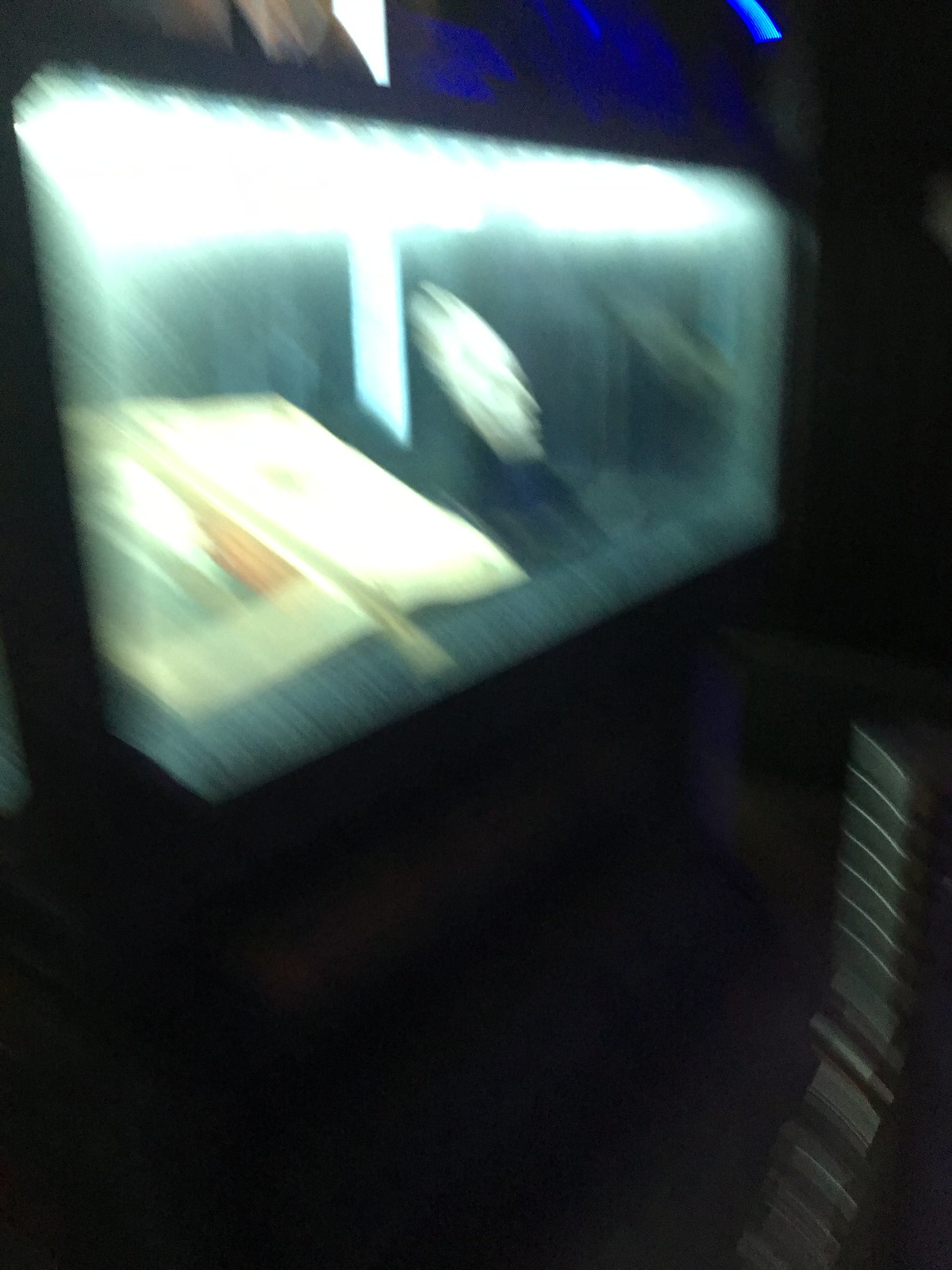The image captures a scene that is profoundly blurry, indicating that the photo was taken in the midst of movement, causing the camera to jolt. The overall atmosphere is very dark, with the majority of the image shrouded in shadow, making it challenging to discern specific details. However, a noticeable feature is located towards the top left corner: a bright rectangular section emitting a light that's predominantly white with a subtle blue hue. This light could resemble a fish tank, an aquarium, the interior of a computer, or possibly a television screen, given its rectangular shape and the way it illuminates surrounding objects.

Inside this lit rectangle, various shapes and colors are visible, including light yellows, different shades of blue, and greenish-blue hues, contributing to the assumption that some kind of electronic or illuminated device is present. Above this lit area, there are pronounced saturated blue smudges whose origins are unclear. Additional indistinct shapes and a white area also appear within the illuminated rectangle, adding to the mystery of what this section might contain.

The rest of the image is cloaked in varying intensities of darkness, creating multiple shadowy regions. In the bottom right corner, there appears to be a formation that resembles a tall stack of books. However, it might also be an optical illusion caused by the interplay of light and the camera's jolt, resulting in the appearance of numerous lines. The overall composition is characterized by its dark, obscure nature, punctuated by a singular, enigmatic source of light.